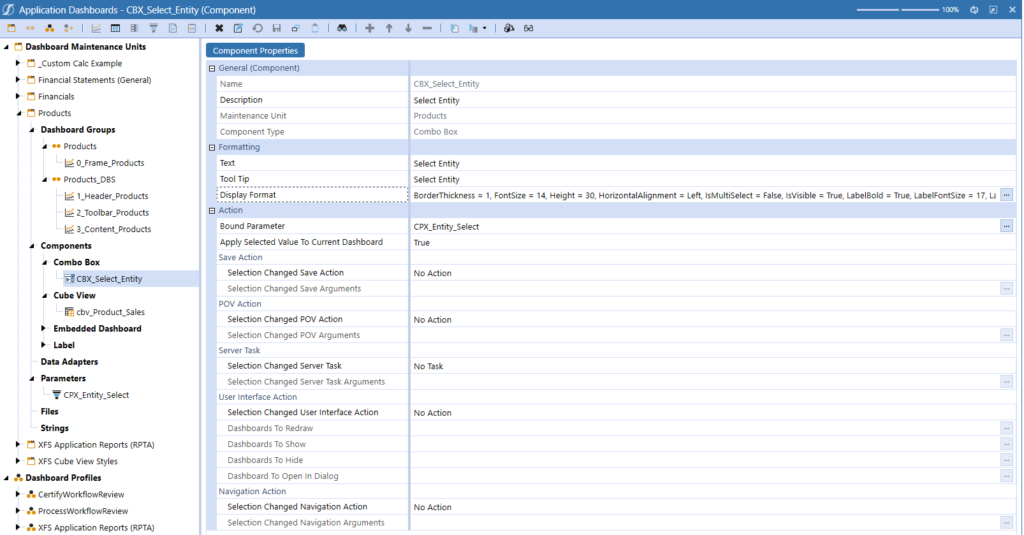In this image, we see a screenshot of a website. At the top left, the header displays "Application Dashboards" followed by "cbx_select_entity (Component)" in white text. To the right of the header, there are two dashed lines and four icons.

On the left-hand side of the screenshot, there is a vertical menu titled "Dashboard Maintenance Units," featuring a list of options that are organized into categories. Some of these categories are expanded to reveal sub-files listed in gray text.

To the right of this menu, there are three sections named "General Component," "Formatting," and "Action," each containing written text in either light gray or black. These sections are organized vertically, with "General Component" at the top, followed by "Formatting," and then "Action."

On the far right-hand side, a larger section is displayed, and it is the most prominent among all sections. This section is titled "cbx_entity_select" and contains multiple entries such as "No Action," "No Action," "No Task," "No Action," and "No Action." Each entry is spaced vertically a few lines apart.

The entire layout has a white background, with the exception of a few columns that are highlighted in a light gray background.